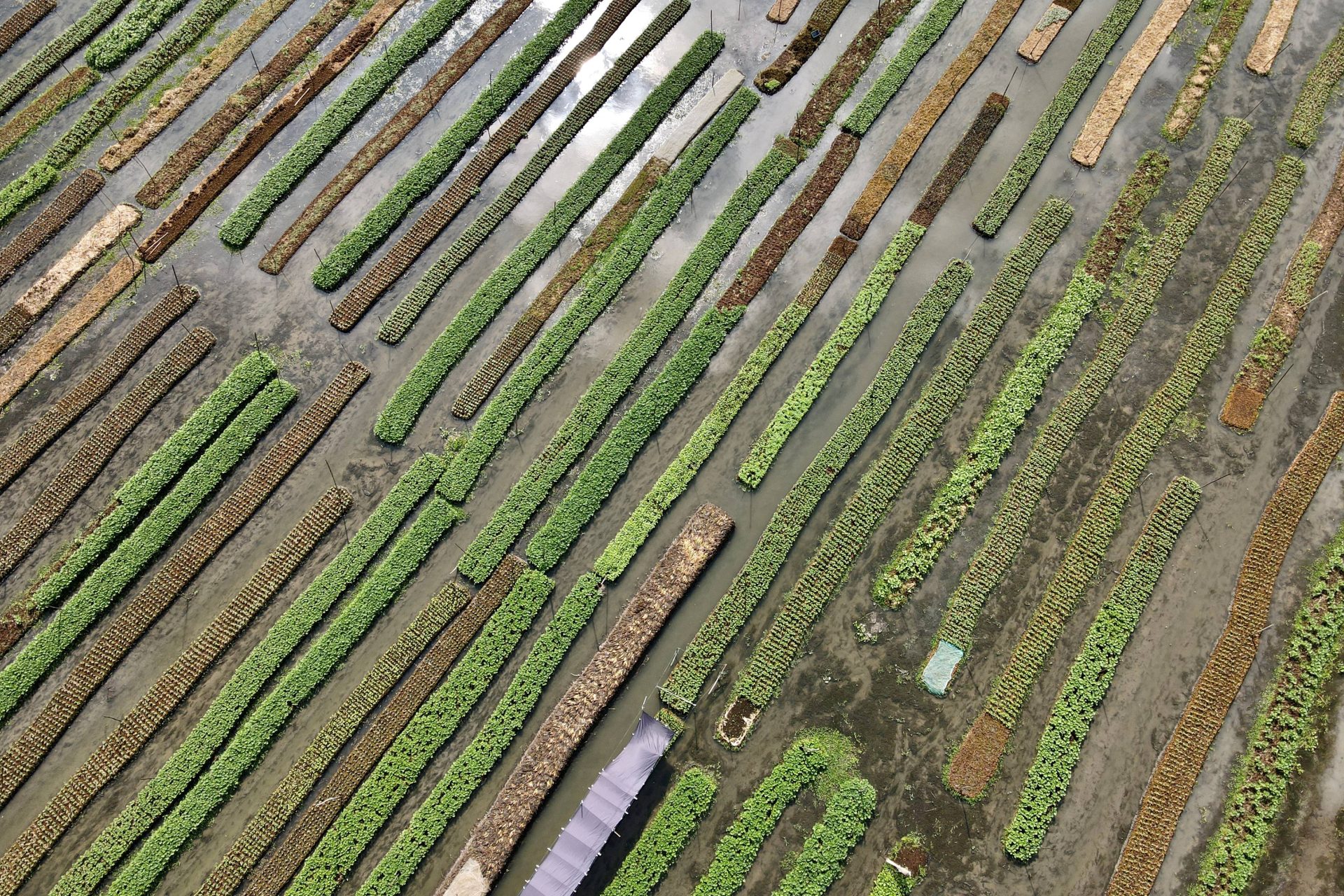The image shows an aerial view of a unique, wet farming area featuring long, skinny strips of greenery and bare soil, which look like floating pieces of lawn. These strips are in a body of water, as indicated by the reflection of the sky, sunlight, and clouds visible on the surface. The vegetation varies in color from light green to dark green, and some strips are brown, indicating different stages or types of crops. There are sticks protruding from the ends of these strips, suggesting some form of support or markers. The overall scene is bathed in daylight, with the water and muddy banks clearly visible between the rows of crops.